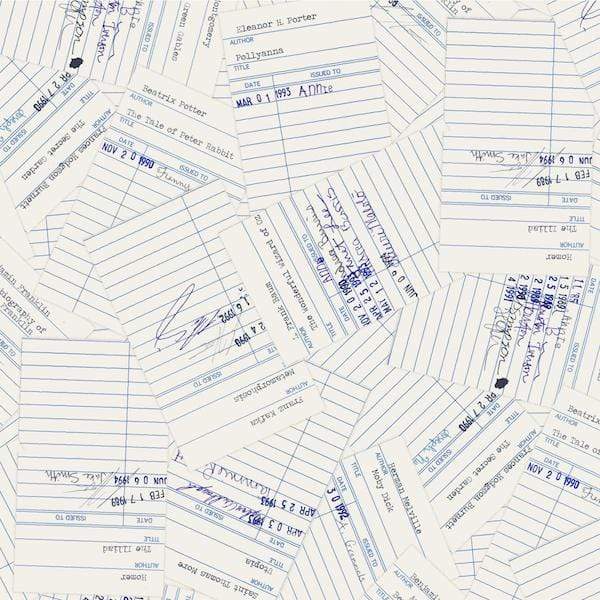The image depicts a chaotic assortment of library checkout slips—small index card-sized pieces of paper—scattered and overlapping in various directions, including upside down, sideways, and at angles. These white cards feature blue horizontal stripes and a single vertical stripe that divides sections labeled for the date and who the book was issued to. At the top of each card, there's a designated space for the author and the title of the book. The dates appear stamped with a mechanical hand stamp, and the names of the borrowers are handwritten. Among the visible cards, one lists "Beecher X. Potter" as the author of "The Tale of Peter Rabbit" with a stamped date of November 20th, 1990. Another card shows "Eleanor H. Porter" as the author of "Pollyanna," with a stamped date that's either March 01, 1993, or 1995, and a child’s name, Annie, written as the borrower. These slips, likely from a school library, evoke a nostalgic glimpse into the record-keeping practices of past decades.